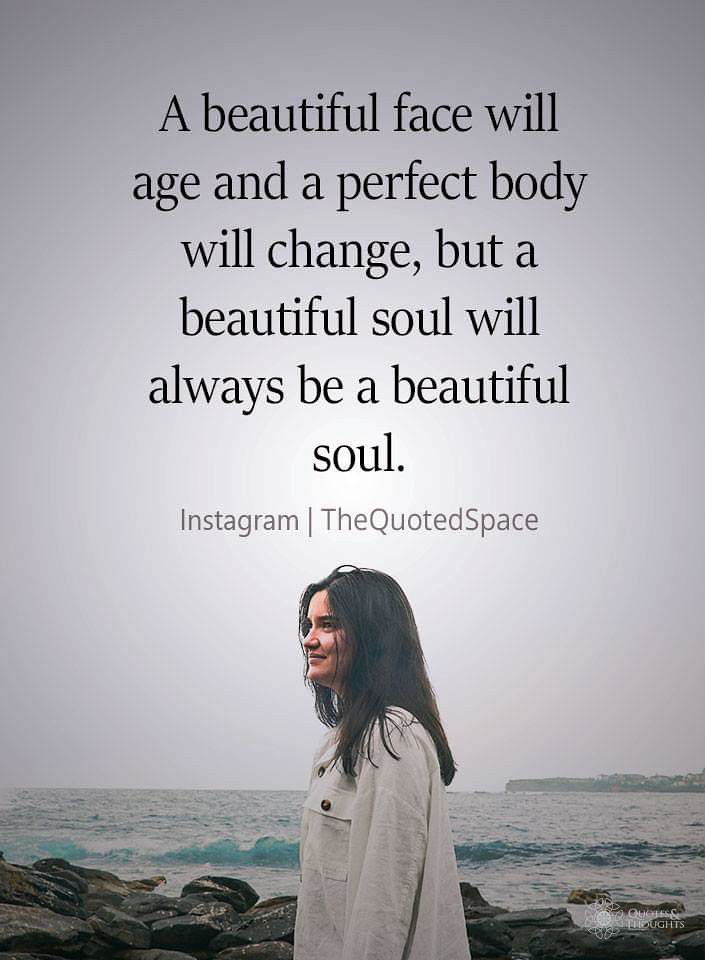In the foreground of this Instagram photo stands a young woman with long, dark hair, viewed from the left side. She is wearing a light tan or gray shirt, standing by the rocky shoreline with the ocean behind her. The sea has gentle waves, and tall trees can be seen in the distance under a gray, overcast sky. Superimposed over the sky is a quote in black text: "A beautiful face will age, and a perfect body will change, but a beautiful soul will always be a beautiful soul." Below the quote, in lighter gray text, it reads, "Instagram / the quoted space."